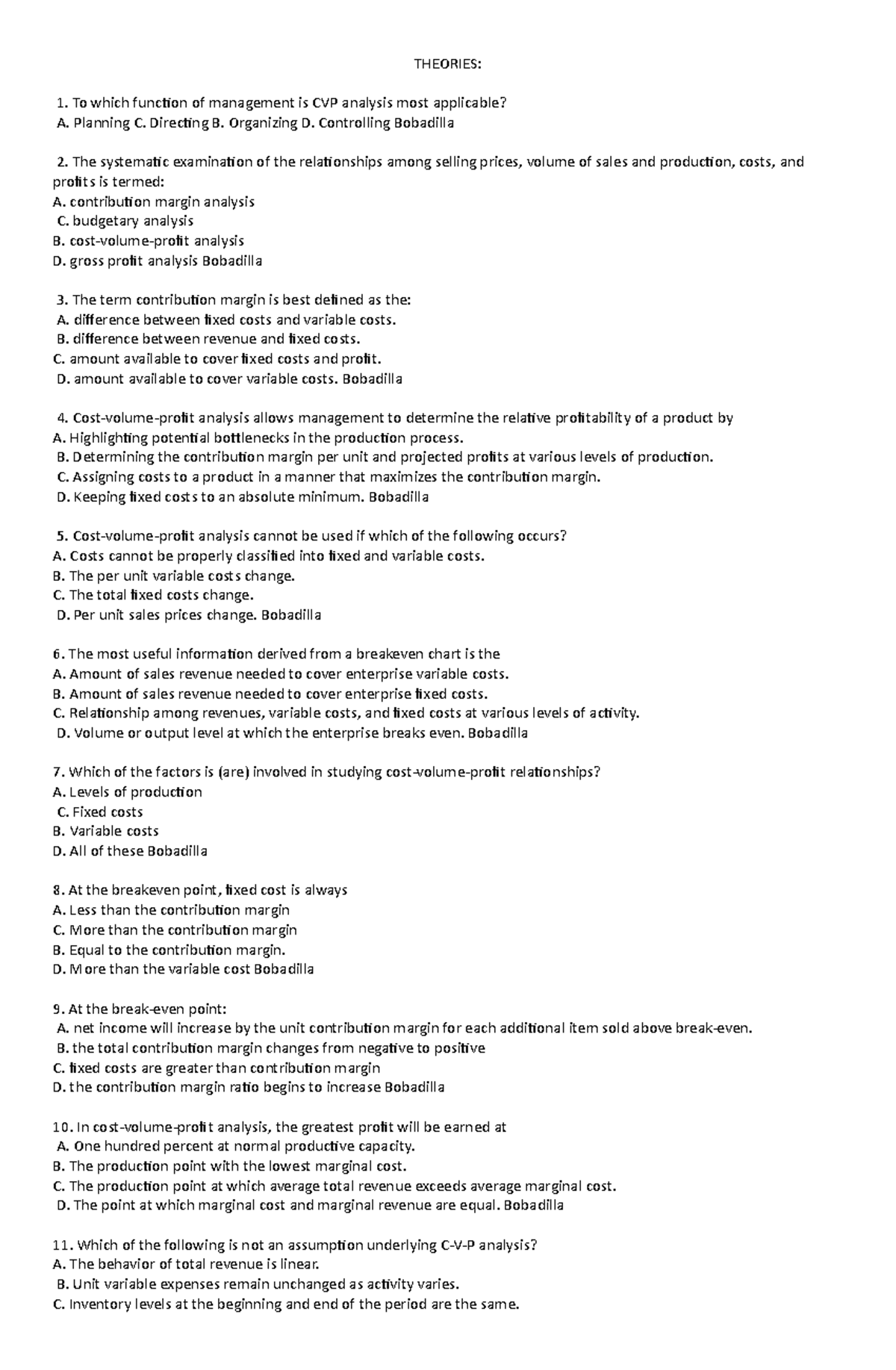The image displays a test focused on theoretical concepts related to management and financial analysis. It's a textual list set against a white background with black text, and is labeled "Theories" at the top. The content consists of a numbered list from 1 to 11, each entry presenting a question followed by four multiple-choice options.

1. **Question 1:** "In which function of management is CP analysis most applicable?"
2. **Question 2:** "The systematic examination of the relationships among selling prices, volume of sales and production, costs, and profits is formed."
3. **Question 3:** "The term contribution margin is best defined as the..."

Each question features four answer choices labeled A, B, C, and D. For example:

- **Question 8:** "At the break-even point, fixed cost is always:"
  - A. Less than the contribution margin
  - B. Equal to the contribution margin
  - C. More than the contribution margin
  - D. More than the variable cost

The format repeats consistently for all eleven questions, making the nature of the document clear as a theoretical examination on management principles and CP analysis.